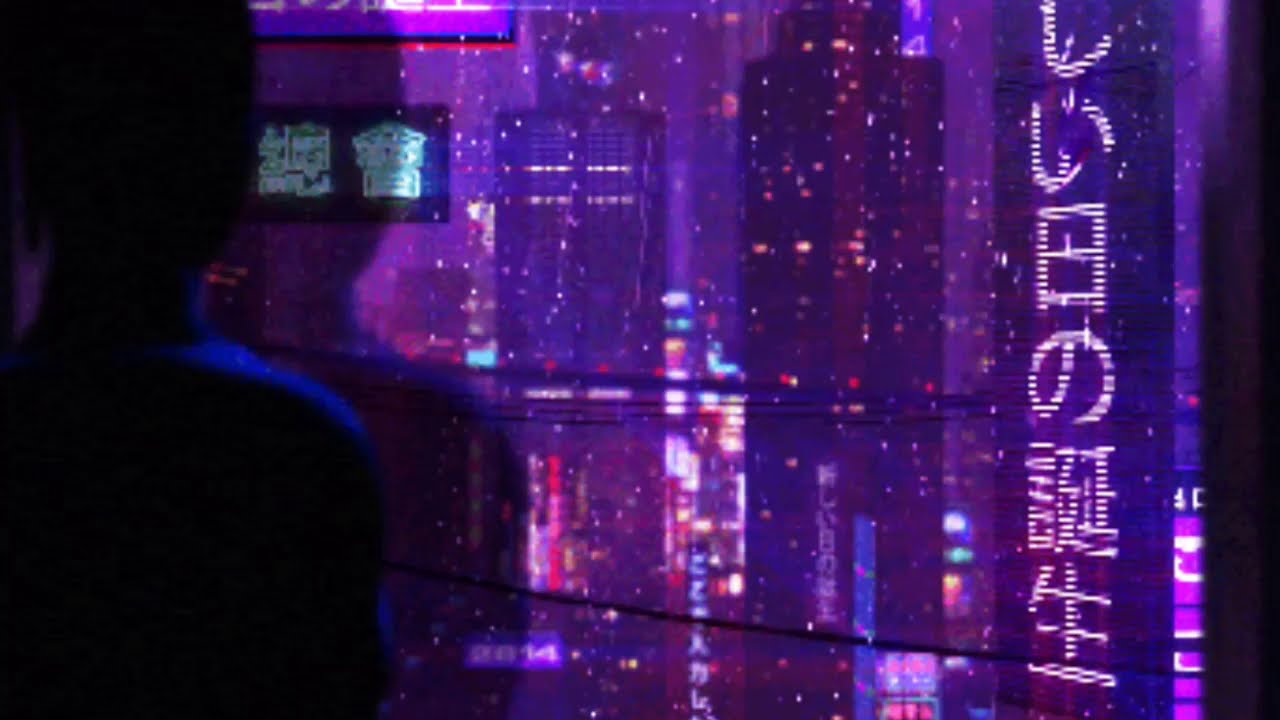This is an evocative nighttime image of an Asian cityscape, likely Chinese or Japanese, viewed through a rain-streaked window. Dominated by hues of purple, with blues, reds, and whites interspersed, the city reveals silhouettes of towering skyscrapers. Some of their windows are faintly lit, creating a mosaic of glowing rectangles against the dark sky. A solitary figure stands to the left, their shadow casting a deeper darkness against the window. To the right of this silhouette, a vertical column adorned with Chinese characters serves as a sign, adding to the enigmatic atmosphere. The overall scene is blurred by the rain, with vibrant reflections dancing on the wet surfaces, blending the colors together in a mesmerizing array.